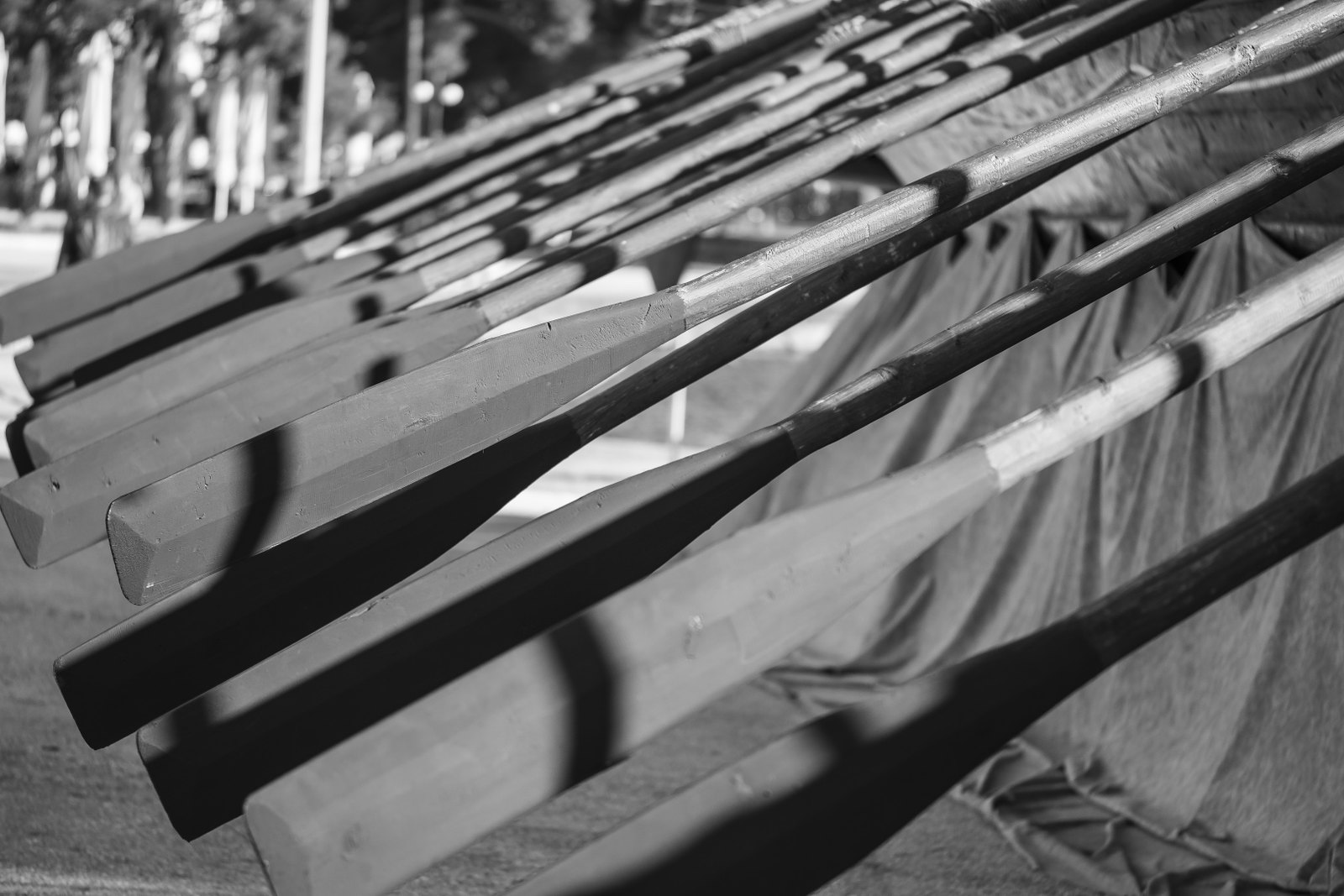This striking black-and-white photo captures a close-up of numerous slender wooden oars, likely for a competition rowboat, with their detailed design featuring a raised edge in the middle and painted flat fanned ends. The oars, all precisely aligned, are suspended mid-air as they rest, suggesting they are part of a large, multi-rower canoe setup. The canoe itself is shrouded in cloth and appears to be elevated or on a platform, possibly for a celebratory display or team recognition. In the background, the blurred outlines of tall trees and a small structure add depth to the scene, while the faint sunlight filters through, casting reflective glints and shadows on the oars. Additionally, there's a hint of activity with the back view of a person walking towards the trees, reinforcing the impression of an outdoor location, potentially a park or schoolyard, setting an ambient scene of calm yet ceremonial significance.